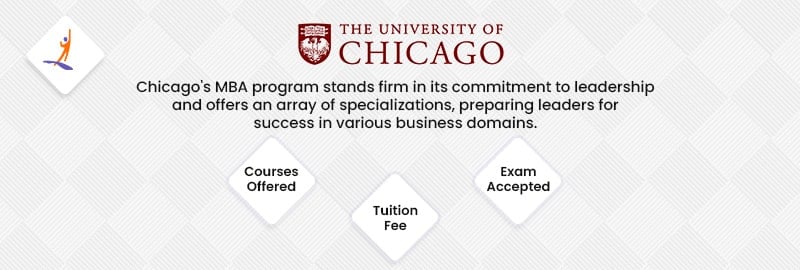The image appears to be a screenshot from the University of Chicago's website, featuring a sophisticated design with a two-toned gray background patterned in diamond or checkerboard shapes. 

In the upper left-hand corner, a highlighted diamond in white depicts an artistic stick figure with a blue head and an orange body, seemingly reaching for the sky, standing on a blue dashed ground.

Centered at the top, the official logo of the University of Chicago is displayed alongside its emblem. Directly below this, a bold black text states: "Chicago's MBA program stands firm in its commitment to leadership and offers an array of specializations preparing leaders for success in various business domains."

Beneath this statement, three white-highlighted diamonds likely serve as clickable buttons, labeled from left to right as "Courses Offered," "Tuition Fee," and "Exam Accepted."

This screenshot represents only the upper section of a comprehensive web page.